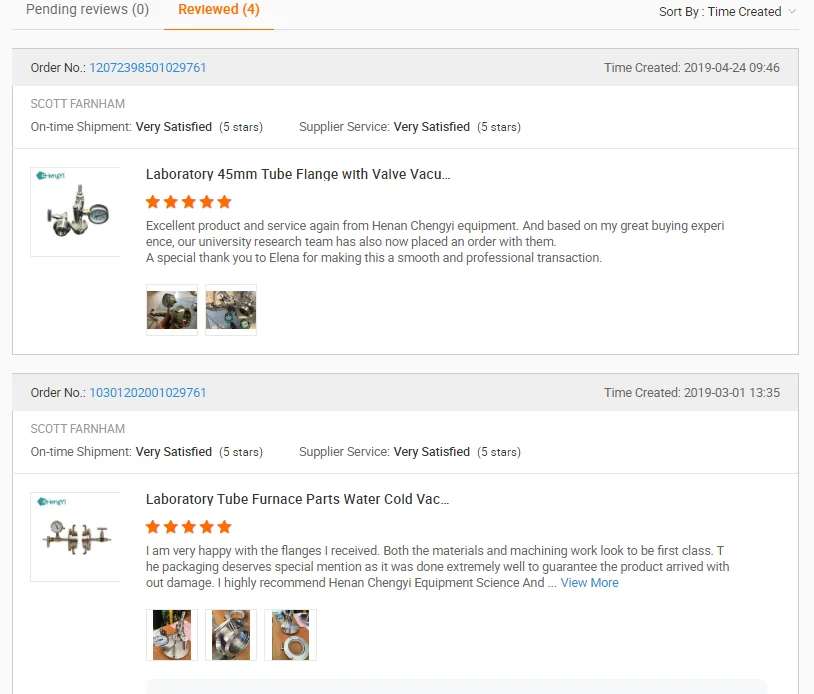The image is a detailed screenshot from a website that summarizes order reviews. 

At the very top, there's a banner displaying review statuses: "Pending Reviews" with a count of (0) and "Reviewed" highlighted in orange with a count of (4). To the right, a sorting option labeled "Sort by" followed by "of: Time Created" with a drop-down menu is available.

Below this main banner, there are two review entries. 

**First Review:**
- **Order Number:** 1-207-2398-501029761
- **Time Created:** 2019-04-24 at 09:46
- **Customer:** Scott Farnham
- **Shipment Type:** One-Time Shipment
- **Customer Satisfaction:** Very Satisfied (5 stars)
- **Supplier Service:** Very Satisfied (5 stars)
- **Item:** Laboratory 45MM2 flange with Valve
 
**Second Review:**
- **Order Number:** 10301202001029761
- **Time Created:** 2019-03-01 at 13:35
- **Customer:** Scott Farnham
- **Shipment Type:** One-Time Shipment
- **Customer Satisfaction:** Very Satisfied (5 stars)
- **Supplier Service:** Very Satisfied (5 stars)
- **Item:** Laboratory two furnace parts: Cold Water, Cold Vacuum

Each review includes detailed feedback from the customer, Scott Farnham, indicating high satisfaction with both the shipment and supplier services.